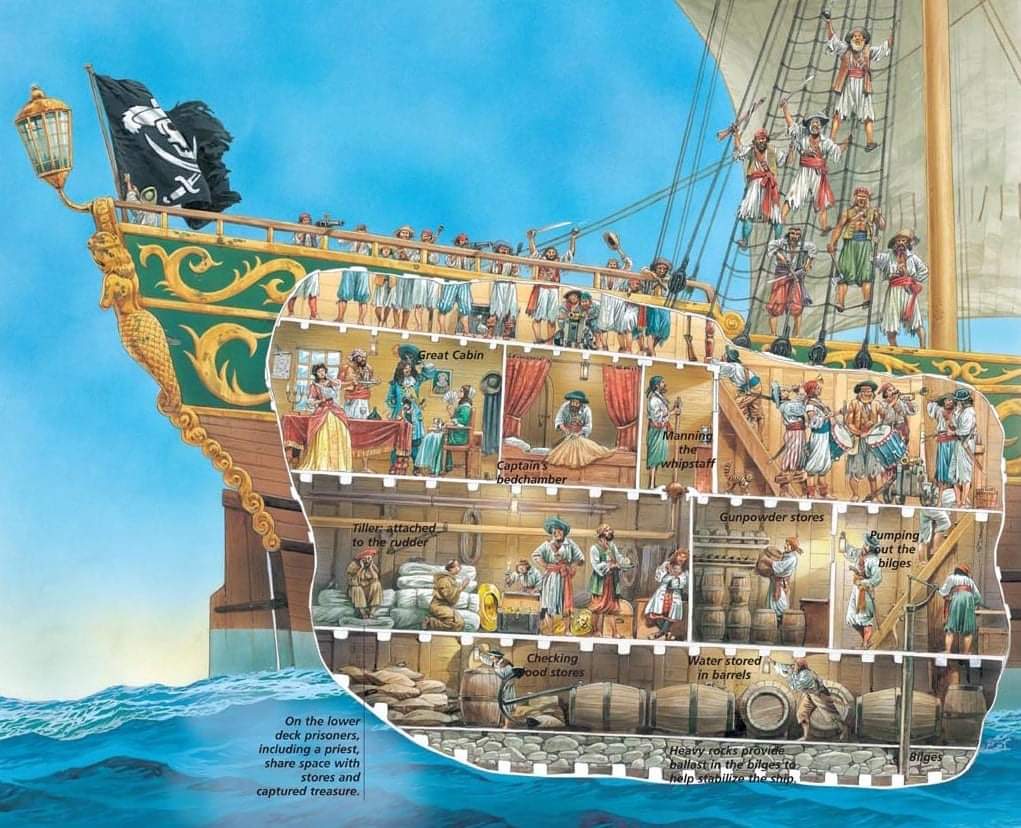This detailed cross-section illustration of a pirate ship from an illustrated children's book reveals the bustling life aboard a typical pirate vessel. At the very top, the ship is adorned with a classic Jolly Roger flag—a black flag featuring a skull wearing a pirate's hat with two crossed swords underneath. On the top deck, a group of stereotypical pirates, some brandishing pistols and other weapons, are engaged in various activities. Some are climbing the sail netting, perhaps shouting or singing, adding to the chaotic yet vibrant scene.

The upper-right section of the ship shows the great cabin, where the captain appears to be entertaining two women while another man serves food. Adjacent to this is the captain's bedchamber, where an underling is busy making the bed. Below these quarters, another pirate is manning the whip staff, responsible for steering the ship. Further rooms include the tiller attached to the rudder, which is crucial for navigating the vessel.

On the lower deck, prisoners—including a priest—are held alongside stores and captured treasure. Nearby, someone is seen checking wood stores and water barrels, ensuring the ship's supplies are in order. At the very bottom, in the bilges, heavy rocks provide ballast to stabilize the ship, while crew members pump out excess water to keep the ship afloat. The gunpowder storage is also located here, with barrels full of gunpowder being carried by a pirate. The scene vividly captures the dynamic and often harsh life of pirates, filled with various duties and the ever-present threat of danger.